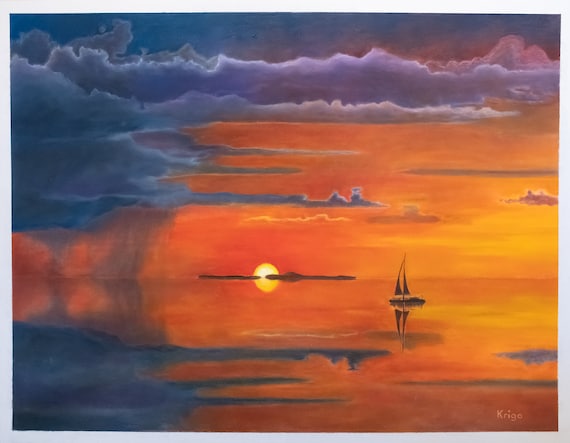This serene painting captures a sailboat with two dark sails gliding across tranquil waters during a mesmerizing sunset. The sky and sea are bathed in vibrant shades of orange, accented by murky, dark clouds of gray, purple, and blue. The setting sun, glowing bright yellow, is positioned in the middle background, partially obscured by an indistinct land structure, casting dramatic lighting throughout the scene. The water reflects the brilliant colors of the sky, creating a nearly symmetrical visual effect between the two. A faint horizon line separates the mirrored expanse of sky and sea. The painting, likely signed "KRIGO" in light white in the bottom right corner, features a subtle white border that suggests it is a framed work of art, adding a refined touch to this captivating maritime scene.